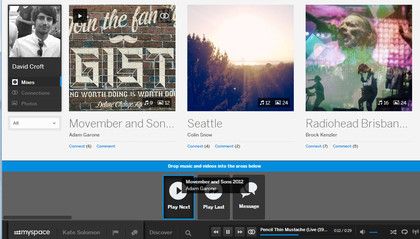The image consists of four distinct sections arranged at the top. At the beginning, there are four smaller images. The first one features the text "David Croft" in white, and below it, "Doing the Family Gifts" is also written in white. Further down, it says "Seattle" accompanied by an illustration of the sun and brown trees. There's a musical note somewhere in this section with the number "24" in white, but the rest of the text is unreadable, even upon zooming in.

The second section displays the word "Radiohead" with partial text "Briss B-A-N..." followed by an ellipsis, set against a blue background. Below this, there are three people shown performing on stage. There's more white text that reads "Drag or Drop Music," but the remaining words are too blurry to decipher.

The third section consists of three dark gray rectangles, each containing some text in white. The first rectangle, highlighted in blue, reads "Play Music." The second seems to say "Playlists" or something similar. The third rectangle possibly says "Manage," but this is not clear.

At the bottom, the text "MySpace Kate Solomon" appears in white, possibly indicating the person's name. Next to it, there is a white flag and a white text box, although the purpose of these elements is unclear.